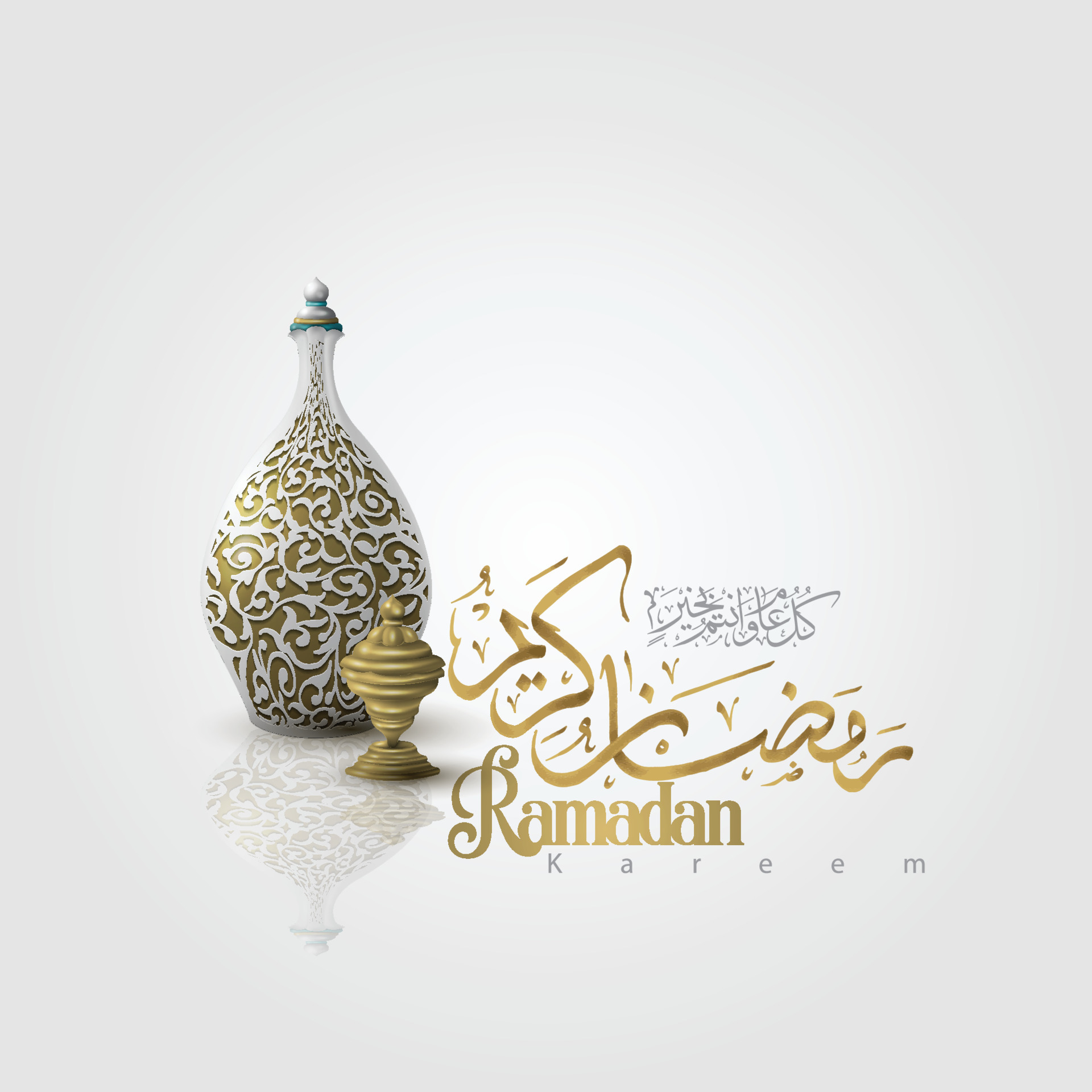The image features two vases set against a stark white background. The vase on the left is tall and slender, characterized by an elegant round shape at its body, which tapers into a narrow neck with a round top. This vase is primarily bronze with intricate white floral patterns adorning its surface, capped with a silver lid embellished with blue lines. Positioned next to it, on the right, is a smaller, diamond-shaped vase, entirely gold with a more condensed and rounded form. Above this smaller vase, there is intricate Arabic calligraphy in gold, and below it, the words "Ramadan" in prominent gold lettering, followed by "Kareem" in smaller silver letters. Additional foreign text, rendered in silver and gold, decorates the space above the smaller vase, contributing to the overall festive and religious theme of the artwork.